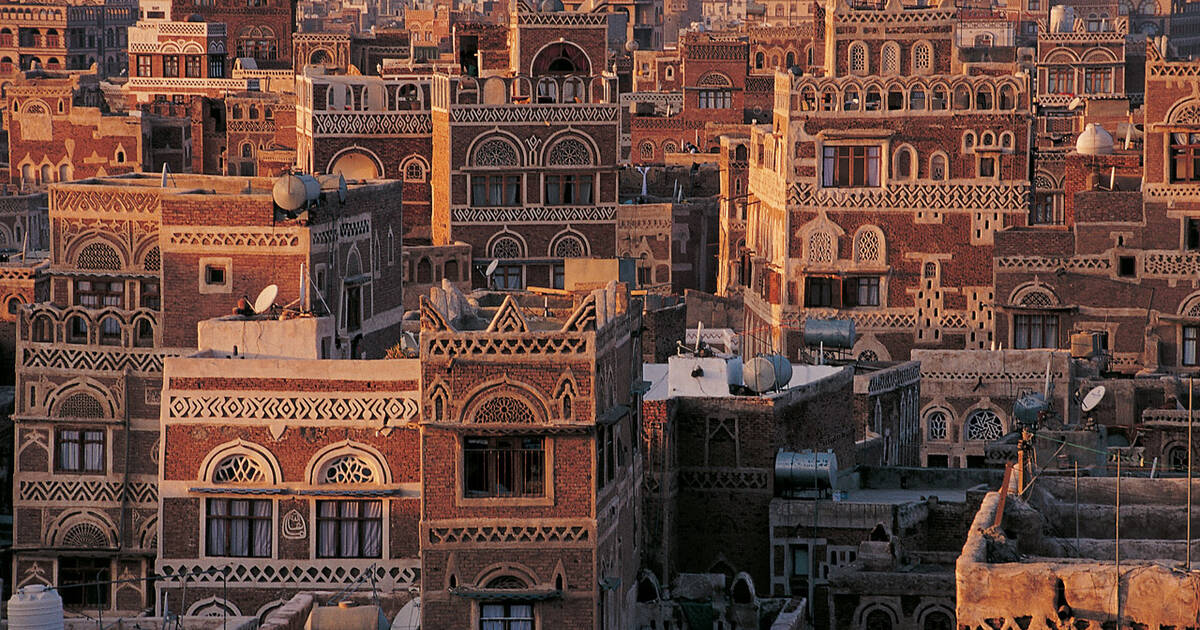A rectangular photograph captures a sprawling cityscape that stretches to the horizon, filled with an array of multi-storied, rectangular, and square buildings. All the buildings share a distinct aesthetic with red brick exteriors and tan-colored trimmings and decorations, reflecting a consistent architectural style that hints at a Middle Eastern influence. As the orange hues of the setting sun cast a warm glow over the city from the top left corner of the image, the buildings' flat roofs are adorned with small decorative railings and dotted with round metal satellite dishes pointing upwards. Additionally, many of the buildings feature clothing wire hangers and electric poles, adding to the urban texture. The photograph is oriented horizontally, with the top and bottom edges being twice as long as the sides, emphasizing the vastness of the city view captured from a high vantage point.